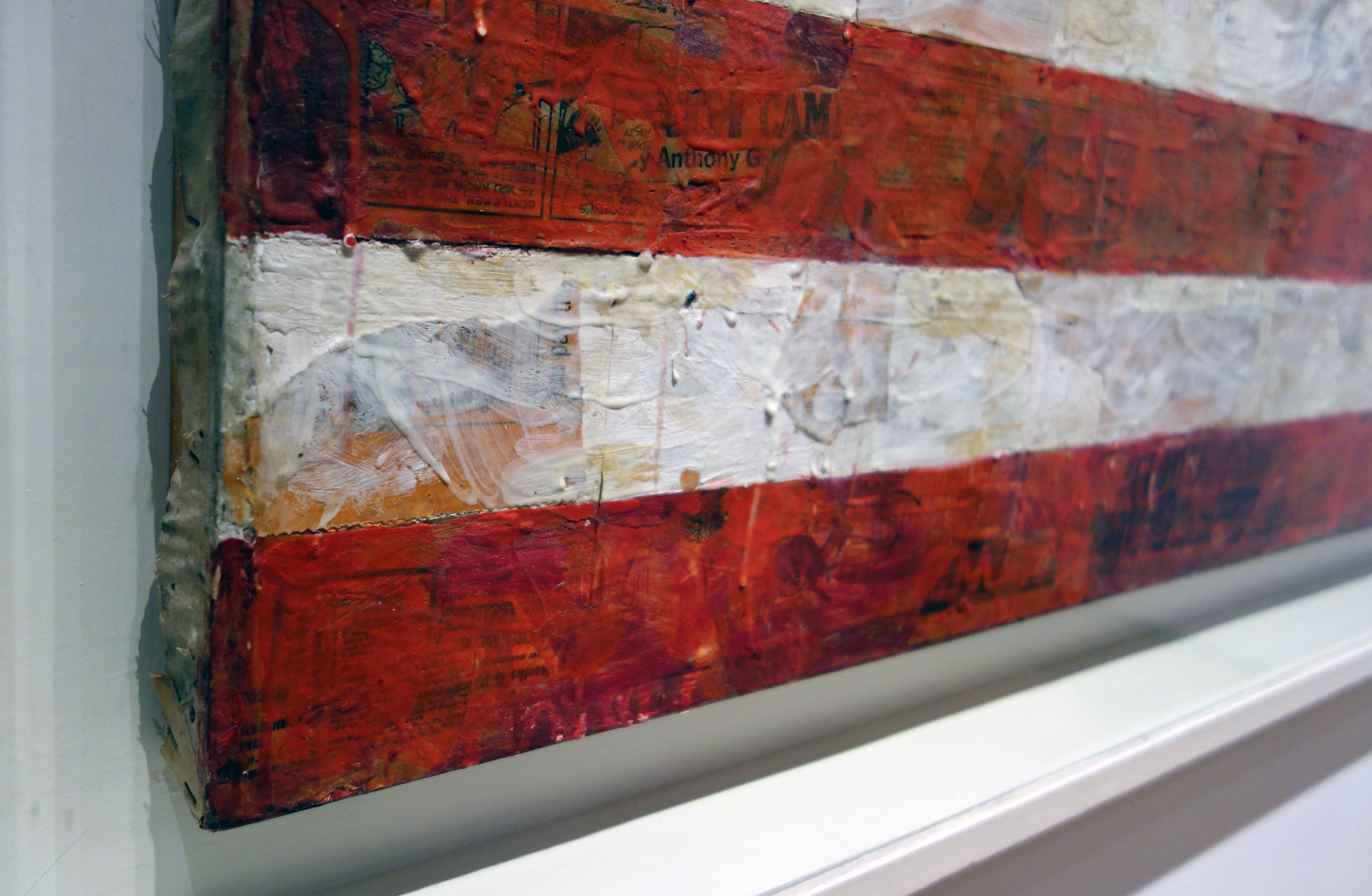The image depicts a three-dimensional art piece affixed to a white wall. The art consists of horizontally stacked boards painted with alternating red and white stripes, resembling a segment of the American flag. However, the paint is applied unevenly, revealing bits of the brown board and underlying layers of black text and newspaper clippings. Near the top edge, bubbles of paint further emphasize its rough and textured appearance. This dimensional creation extends outwardly, adding depth to the artwork, and is supported by a thin ledge or short shelf protruding from the wall, contributing to the overall striking visual effect.